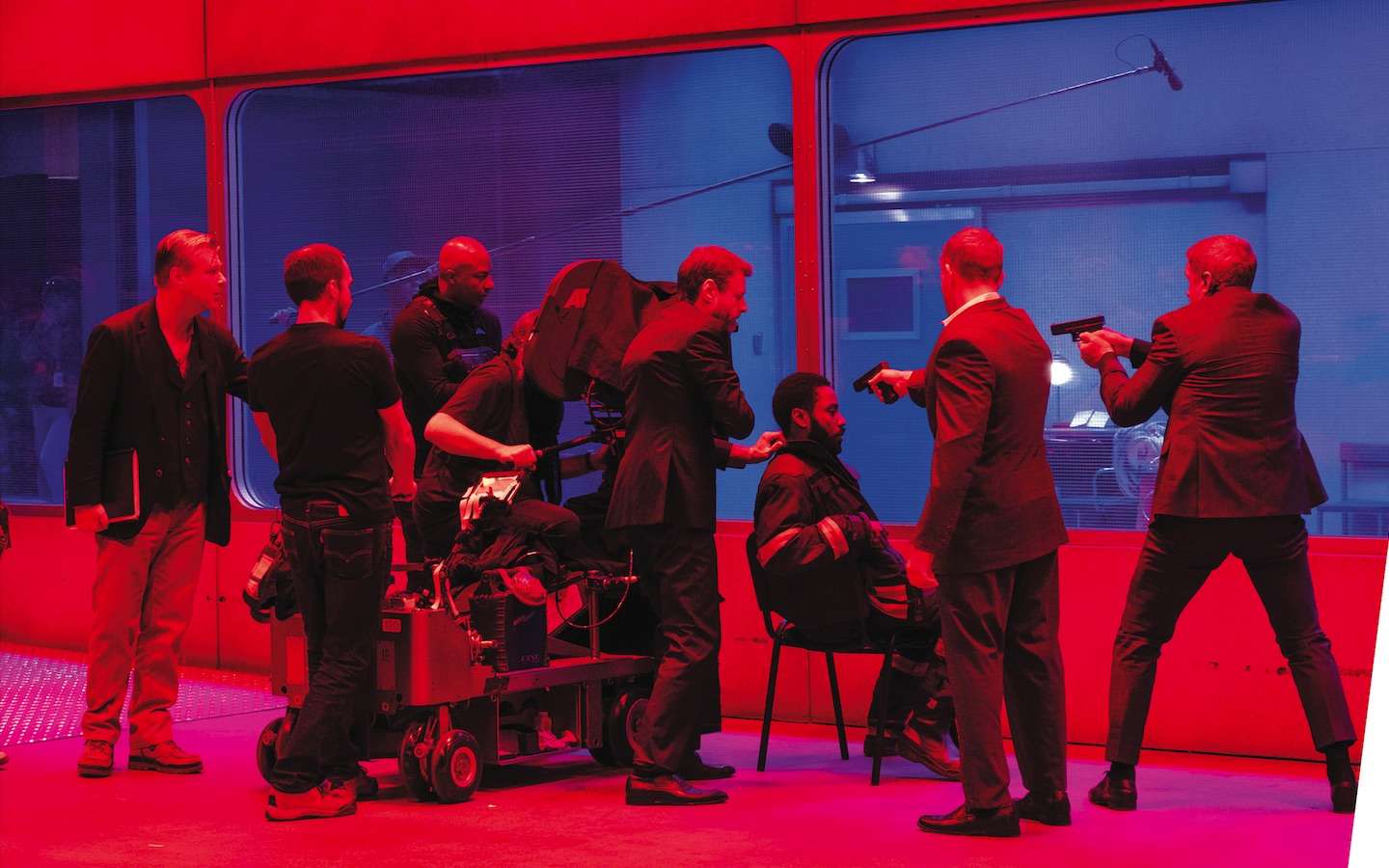This image depicts an intense movie scene in progress, framed under a vivid red tint. At its center, a black man, possibly in a fireman's uniform identified by the striped jacket, is strapped to a chair with a serious expression. In front of him, two men in suits brandish pistols, aiming directly at his head, their backs turned to the camera. To the left, another man places a hand on the seated man's shoulder, seemingly in conversation. Behind this focal point, the active movie set is visible, featuring a cameraman operating a large, wheeled camera positioned to capture the dramatic moment. Additional crew members, including a man in a suit holding what looks like a script or notes in his right hand, stand around, directing or observing the scene. The setup hints at a blue hue outside through three large windows, contributing to the contrasting atmosphere of the shoot. An array of high-placed microphones suggests careful attention to sound capture, further cementing this as a diligent and structured film production environment.